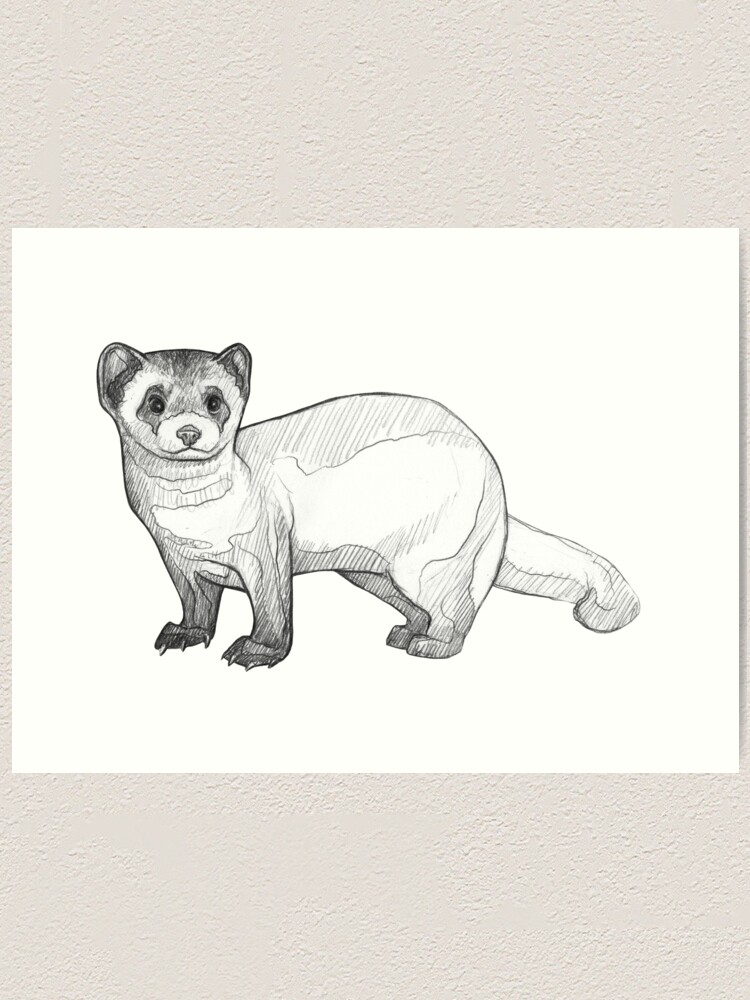The image is a highly detailed illustration, likely created with pencil or charcoal, showcasing a small, rodent-like or mongoose-like creature with a long, slightly curled tail. The animal has a cute and friendly expression, with distinctive patches around its eyes, pointy ears, and a little nose. The creature stands low to the ground on all fours, facing left, giving a clear view of its left side, including its four paws, with claws only on the front ones. The artwork features meticulous hatch lines and shading that enhance its texture, making the animal appear almost lifelike. The illustration is set against a white, slightly grainy background reminiscent of a wall texture, giving the whole scene a clean, stark contrast. The piece of paper holding the artwork is similarly white, blending seamlessly with the wall behind it. This thoughtful composition and attention to detail highlight the skill of the artist.